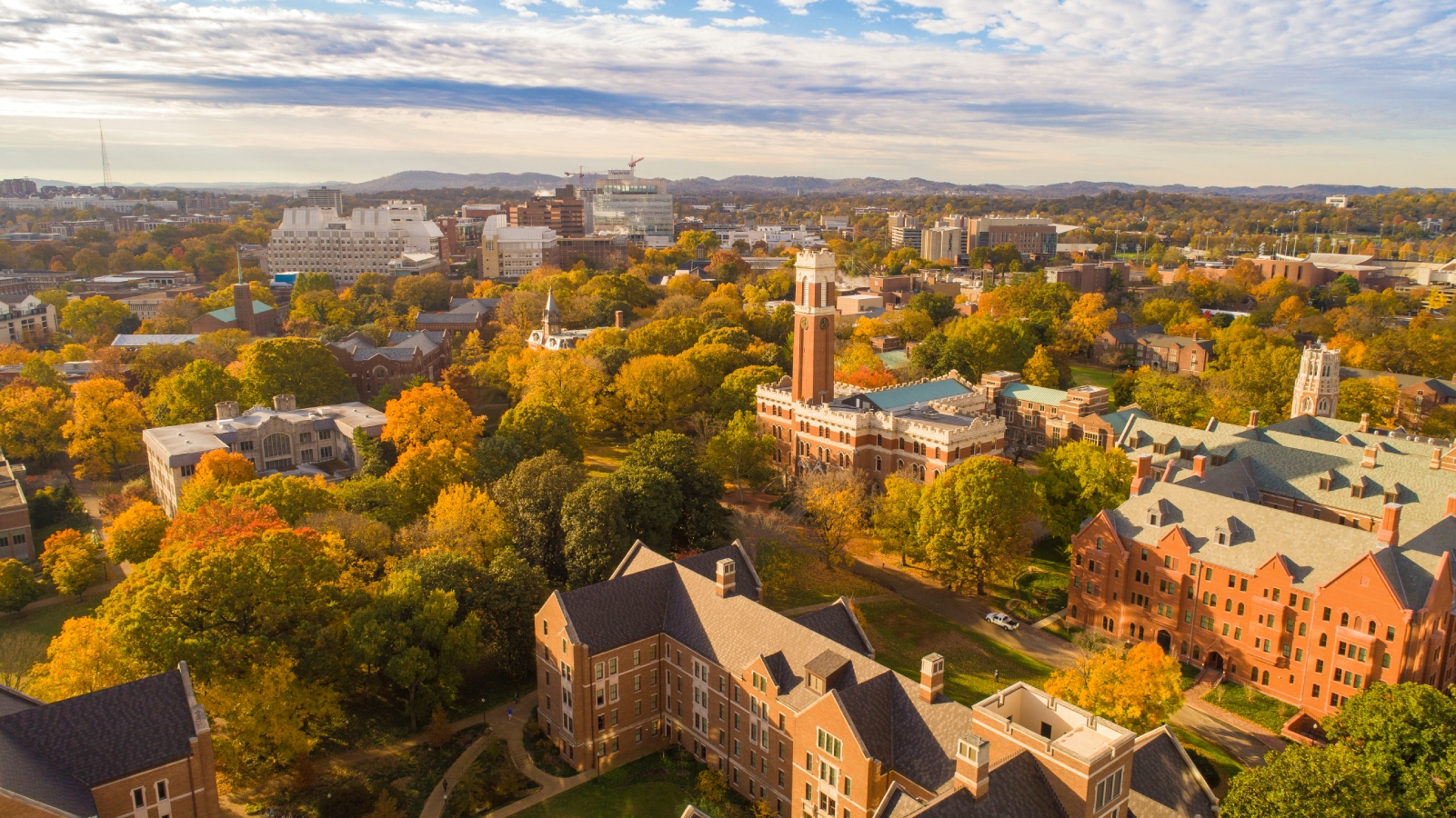This detailed aerial photograph captures a picturesque New England town or college campus during a vibrant autumn day. The top-down view reveals a landscape adorned with abundant fall foliage in shades of green, yellow, and orange, providing a colorful contrast to the historic architecture. The scene is bathed in the golden light of daytime, possibly during golden hour, adding warmth to the image. Prominent in the center is a large brick building with a tall bell tower, suggesting it may serve an institutional purpose such as a university. Surrounding this central structure are numerous multi-story buildings in varying hues of red and brown, some with light-colored roofs that further enhance the variety in the scene. The sky above is a bright blue, dotted with flat oval-shaped clouds, hinting at classic New England weather. In the distance, the landscape gradually rises into low hills or mountains, adding depth and a sense of vastness to the photograph. The cohesive architectural style of the buildings reinforces the impression of a connected community, likely a college campus nestled within this leafy urban environment.